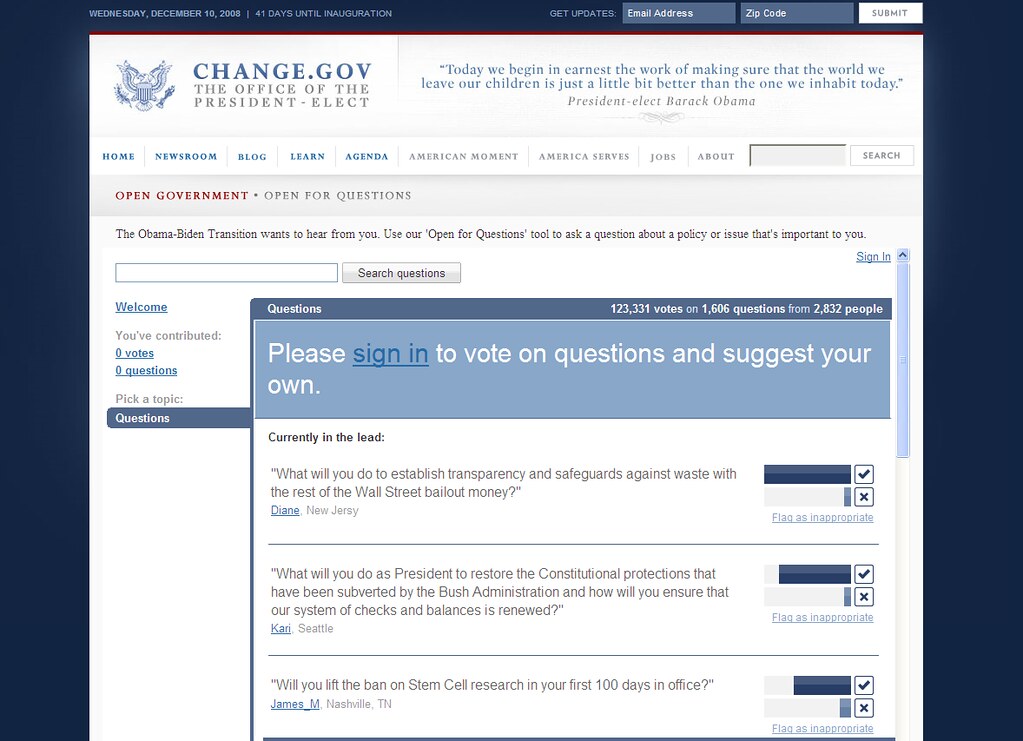This is a detailed screenshot of a tablet or computer displaying the very top section of a website dated Wednesday, December 10, 2008. The header prominently shows "41 days until inauguration," signifying the countdown to the upcoming presidential inauguration. The website featured is "change.gov," representing "the Office of the President-elect." The top section includes a quote from President-elect Barack Obama: "Today we begin in earnest the work of making sure that the world we leave our children is just a little bit better than the one we inhabit today."

A pop-up window appears, urging users to "please sign in to vote on questions and suggest your own." One of the leading questions in this pop-up asks, "What will you do to establish transparency and safeguards against waste with the rest of the Wall Street bailout money?"

The website’s border is in a dark blue hue, and "change.gov" in the upper left-hand corner is displayed in an even darker blue shade.